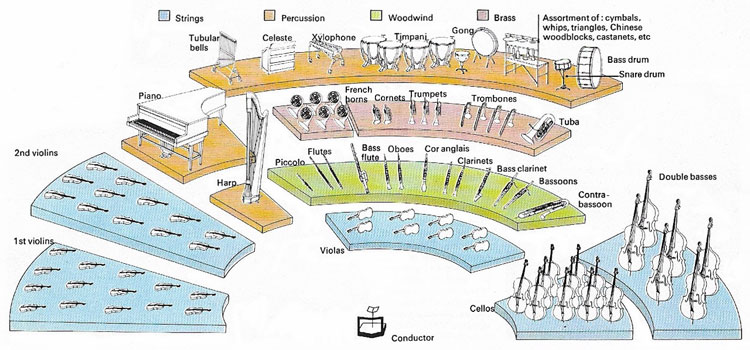This image depicts a detailed, color-coded 3D layout map of an orchestra arrangement, showcasing how various instrument sections are seated and arranged around the conductor, who stands labeled in the center. The layout features a radial and slightly vertical spacing of the orchestra elements, with thick 3D pie wedges representing each instrument section and the number of instruments within them, accompanied by line drawings for visual clarity.

On the right side, the strings section includes cellos and double basses, extending to the violas positioned directly in front of the conductor, followed by the first and second violins. Adjacent to the strings, the woodwinds section comprises piccolo flutes, flutes, bass flutes, oboes, clarinets, bass clarinets, bassoons, and contrabassoons. Behind them, the brass section contains French horns, cornets, trumpets, trombones, and a tuba.

At the uppermost part of the map, the percussion section includes an array of instruments like tubular bells, bass drums, xylophones, and a variety of other percussion instruments. Additionally, there is a large piano and a harp section. The map uses color coding to differentiate sections: string instruments are on blue pedestals, while percussion instruments are on green ones, enhancing the clarity of the orchestra’s seating arrangement.